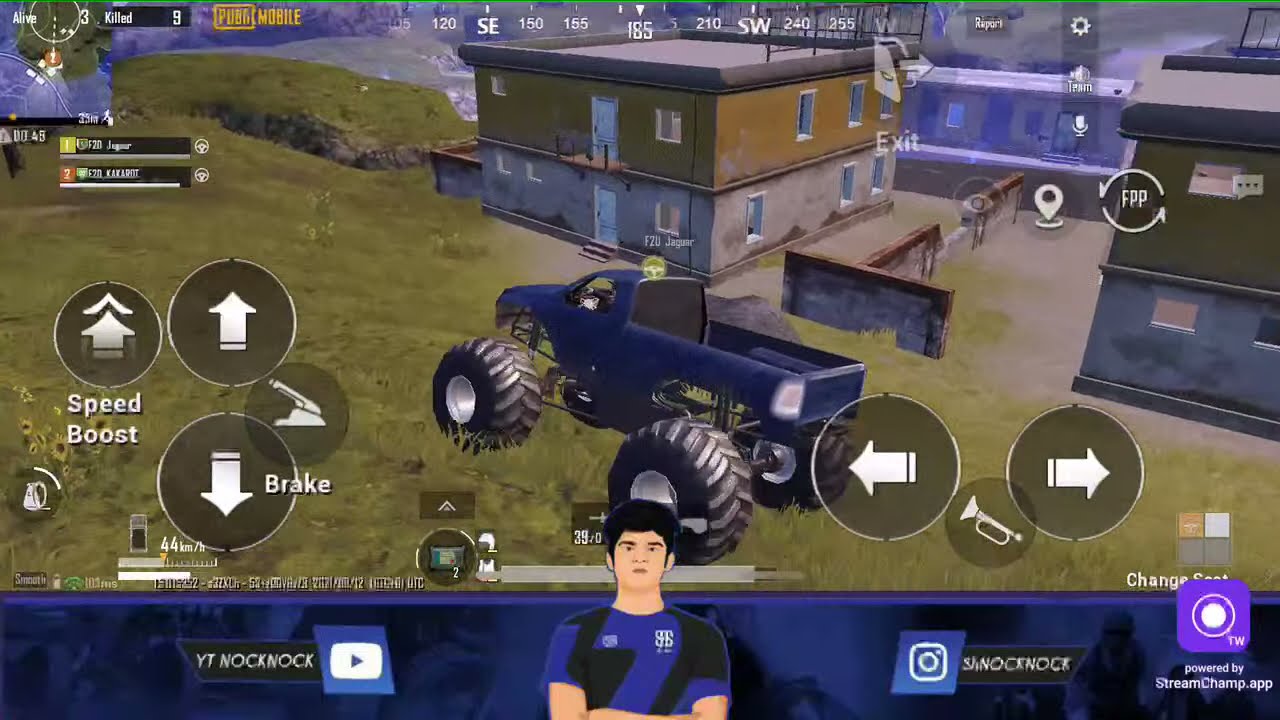This image is a detailed screenshot from a mobile video game, possibly powered by streamchamp.app, as indicated by the purple-logoed text in the bottom right corner. The central focus of the game scene is a blue monster truck with large wheels, navigating a grassy hill, while in the background, there are two older-style, square-shaped apartment buildings with gray concrete lower halves and yellow upper halves with flat, concrete tops and open windows and doors. The top-left corner of the screen displays typical game stats such as "alive" and "killed."

On the left side of the screen are game controls including a brake button and a speed boost button labeled "speed boost." The right side features additional control circles with arrows, and a horn button. At the bottom bar, there are various user interface elements, including links to a YouTube channel and an Instagram account, though the Instagram text is compressed and hard to read. A character figure, possibly the driver, stands to the side of the monster truck. This character appears to be an Asian male with black hair, wearing a black and purple-striped jersey or t-shirt.